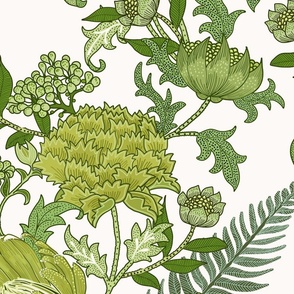The image depicts a detailed square-shaped drawing set against an off-white background, showcasing a variety of green plants and flowers. In the bottom right corner, a frond with narrow, patterned leaves reminiscent of an evergreen plant is present. The drawing features multiple shades of green, including pea green and lighter green hues. Central to the image is a large, bushy flower, resembling an artichoke with segmented leaves. Surrounding it are several other plants: a couple of leafy plants with medium to darker green leaves, and another plant bearing clusters of small, light green berries. Additionally, a prominent flower with petals encircling a dense cluster of small, spherical elements can be seen, with one version of this flower viewed from the side and three others from above. The composition is rich with curly-shaped leaves, varied foliage, and stalks emerging from some plants, creating a lush, intricate botanical scene.